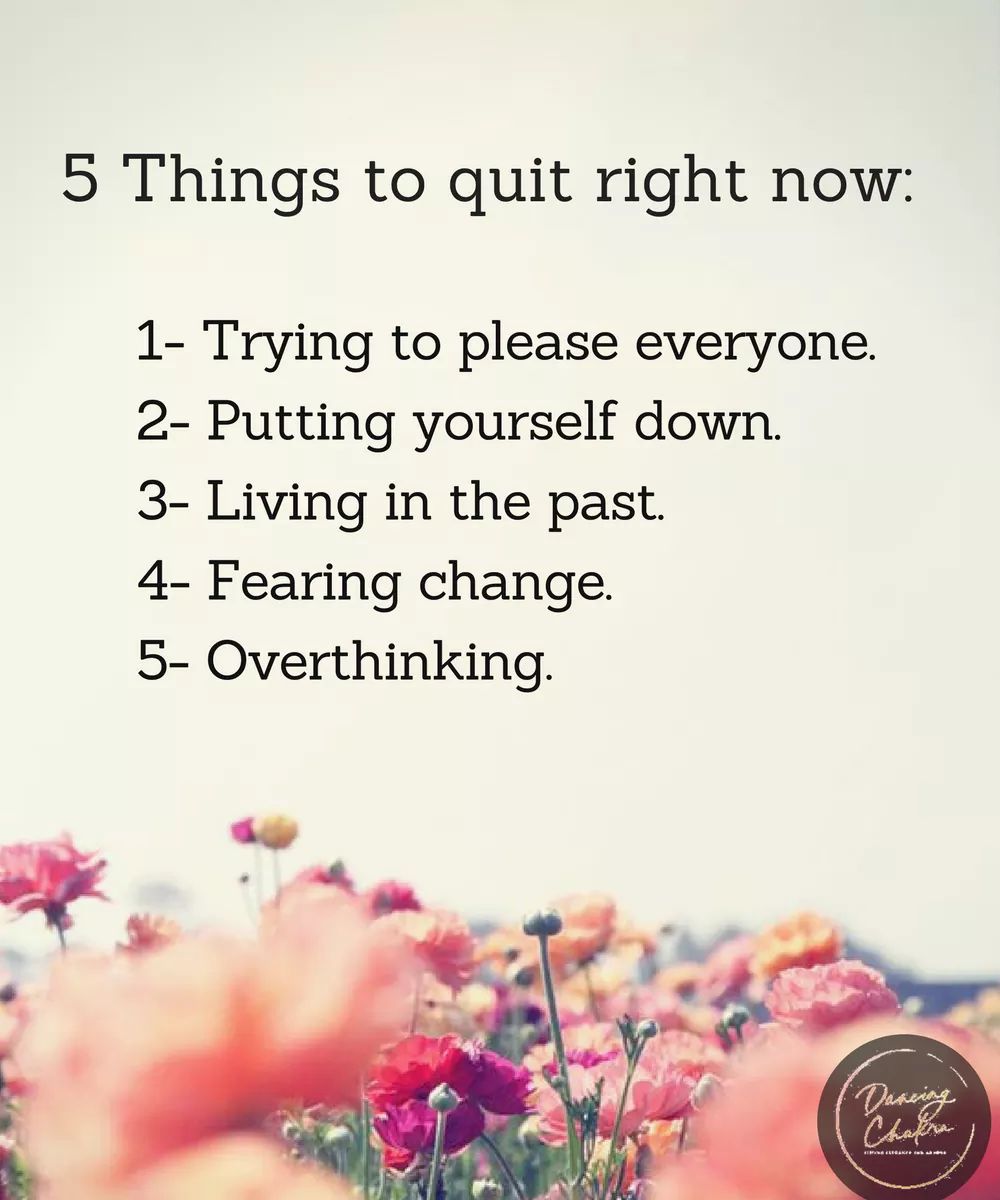The image features a grayish sky-like background and a bottom quarter filled with a field of flowers in varying hues of pink, purple, orangish-yellow, and dark reddish-pink. The flowers closest to the viewer and those in the background appear blurry, while the mid-ground flowers are in clear focus, alongside some unopened pods. Dominating the top three-quarters of the image, black text lists "Five things to quit right now": 1) trying to please everyone, 2) putting yourself down, 3) living in the past, 4) fearing change, and 5) overthinking. In the lower right corner, there is a circular logo in brown with script text that appears to read "Dancing Chakra" in yellow. The overall image has a high level of clarity and brightness, with a clean and reflective tone.